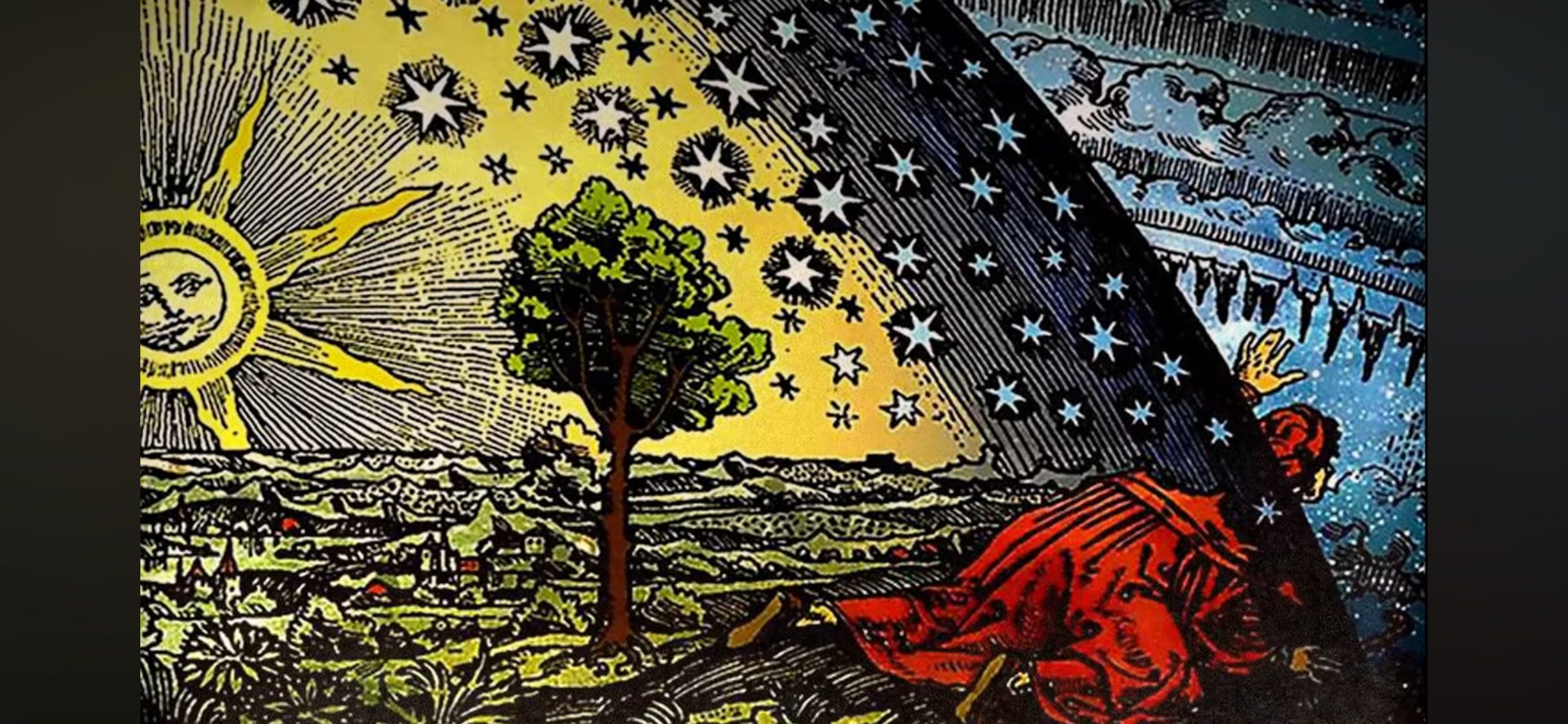The image is a detailed drawing reminiscent of tarot card art, featuring a surreal scene divided into two contrasting realms. At the center is a person, gender ambiguous, wearing a red robe, depicted crawling on their hands and knees. The artwork is split horizontally at the shoulders, with the upper part of the figure crossing into a dark, starry night filled with upside-down clouds and trees, suggesting another dimension or galaxy. On the lower side, the town basks in sunlight with a bright yellow sun and a green tree on the left, contrasting sharply against the cold, dark, blue and black hues, with waves and icicles, of the upper right side. Blue and white stars descend like an arc, adding to the otherworldly atmosphere. This partial view, capturing about one-eighth of an arc or circle, evokes a sense of duality and transition, making the artwork resemble the intricate symbolism found in the Rider-Waite tarot deck, creating a dynamic blend of day and night, reality and fantasy.